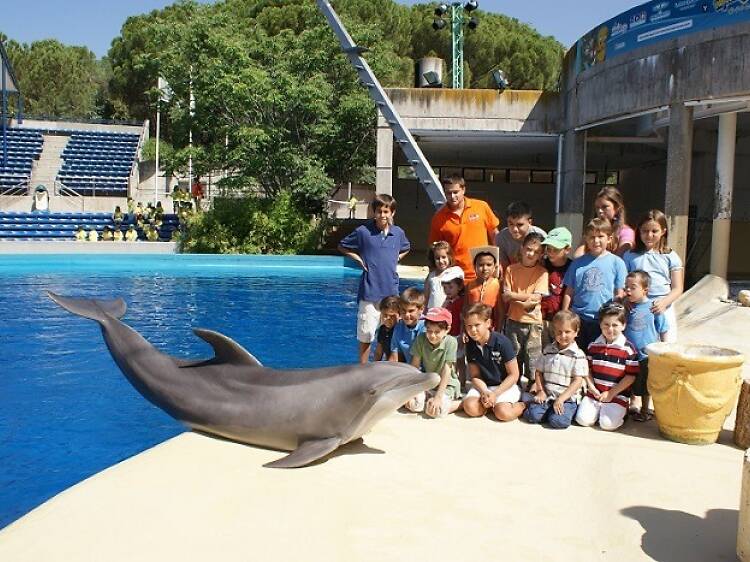In this detailed photograph, we see a group of elementary school children, possibly a first-grade class, gathered in front of a pool. The children are arranged with some standing and others kneeling, forming a multi-row formation. A dolphin has seemingly leaped from the water and now rests partially on the pool's edge, captivating the children's attention. The scene is set in an outdoor marine park, complete with bleachers to the left where a few individuals in yellow shirts are seated. In the background on the right, there are several pillars and a small building, while tall trees and a distinct light blue metal pole equipped with what appears to be four speakers or strobe lights can be seen to the far left. The photograph captures a vibrant array of colors including blue, green, orange, yellow, sage green, dark blue, light blue, beige, brown, white, black, red, and pink, all contributing to the lively and engaging atmosphere of this special event or presentation.